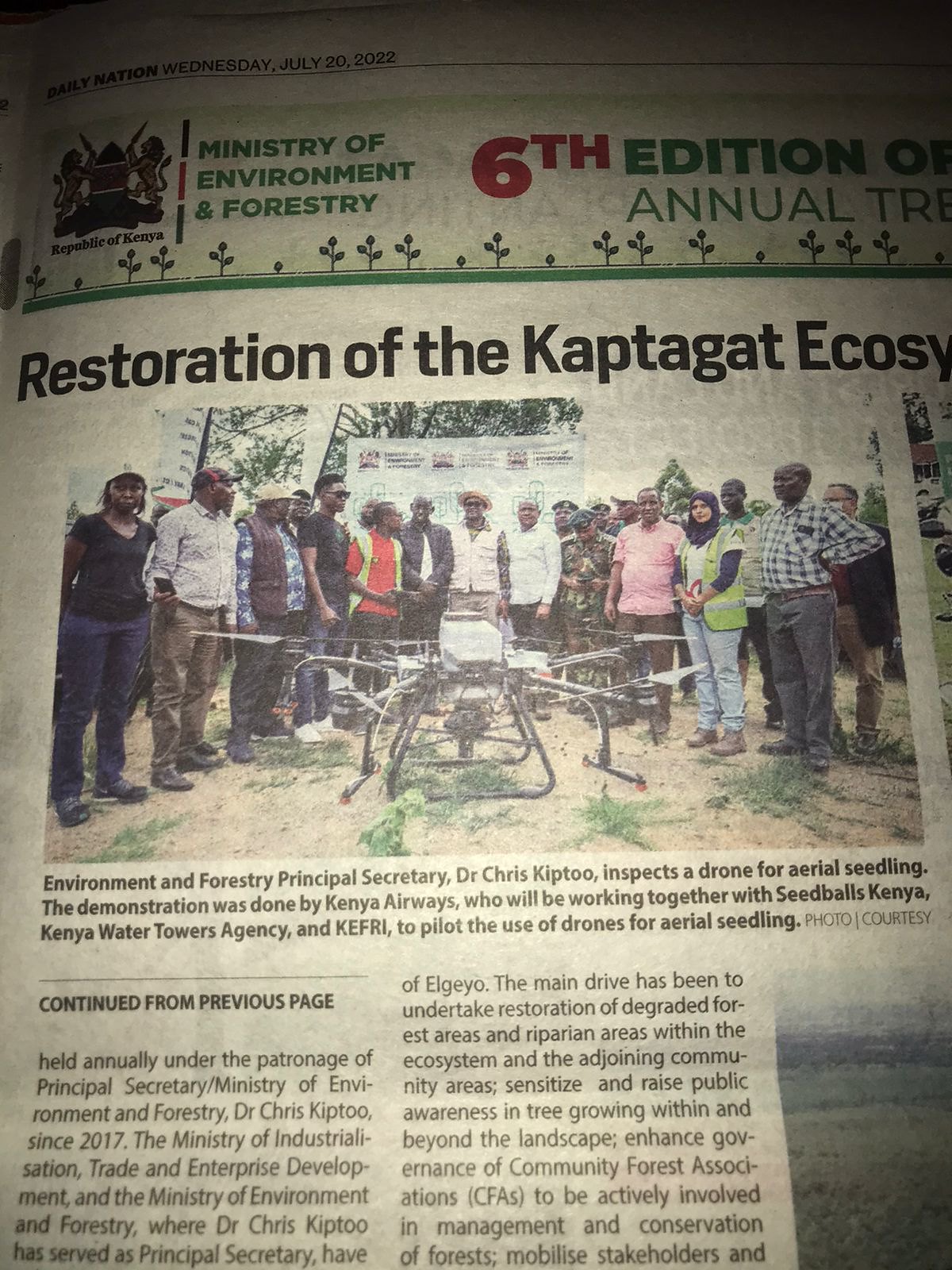This image is a close-up photo of a newspaper or magazine clipping with the header "Ministry of Environment and Forestry, Republic of Kenya, 6th Edition." The main headline reads "Restoration of the Kaptagat Ecosystem." Below this headline is an image depicting around 15 people of varying skin tones, casually dressed, standing in a semi-circle around a large machine. The machine, described as resembling a spider, is a drone being inspected by Environment and Forestry Principal Secretary Dr. Chris Kiptu, as part of a demonstration by Kenya Airways in collaboration with Seed Balls Kenya and the Kenya Water Towers Agency. This demonstration showcases the use of drones for aerial seeding. Behind the group are some trees and a poster, with a caption providing details of the participants and the event. Below this description, an article continues with "Continued from previous page," mentioning the annual patronage of the Principal Secretary of the Ministry of Environment and Forestry.